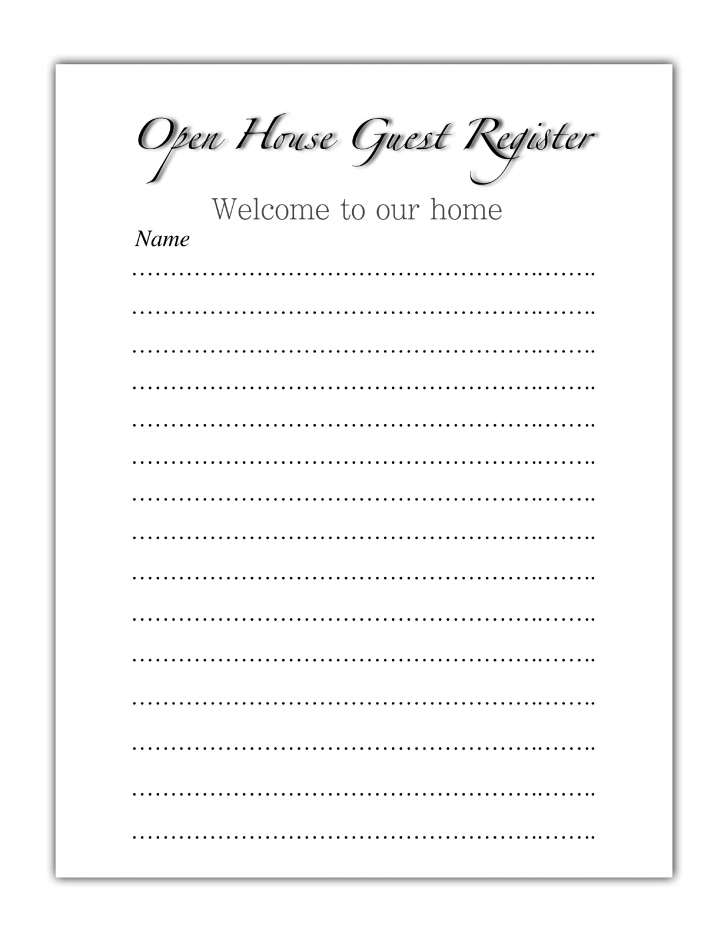This image features a computer-generated rectangular piece of white paper with a delicate black shadowy outline. At the top of the image, in black cursive, it reads, "Open House Guest Register." Directly below this title, in a thinner, non-cursive font, it says, "Welcome to Our Home." Further down on the left side, the word "Name" appears in the same black font. Beneath this, there are 15 black dotted lines arranged in rows, intended for guests to sign their names. The dotted lines extend nearly the entire width of the page, providing ample space for multiple signatures.